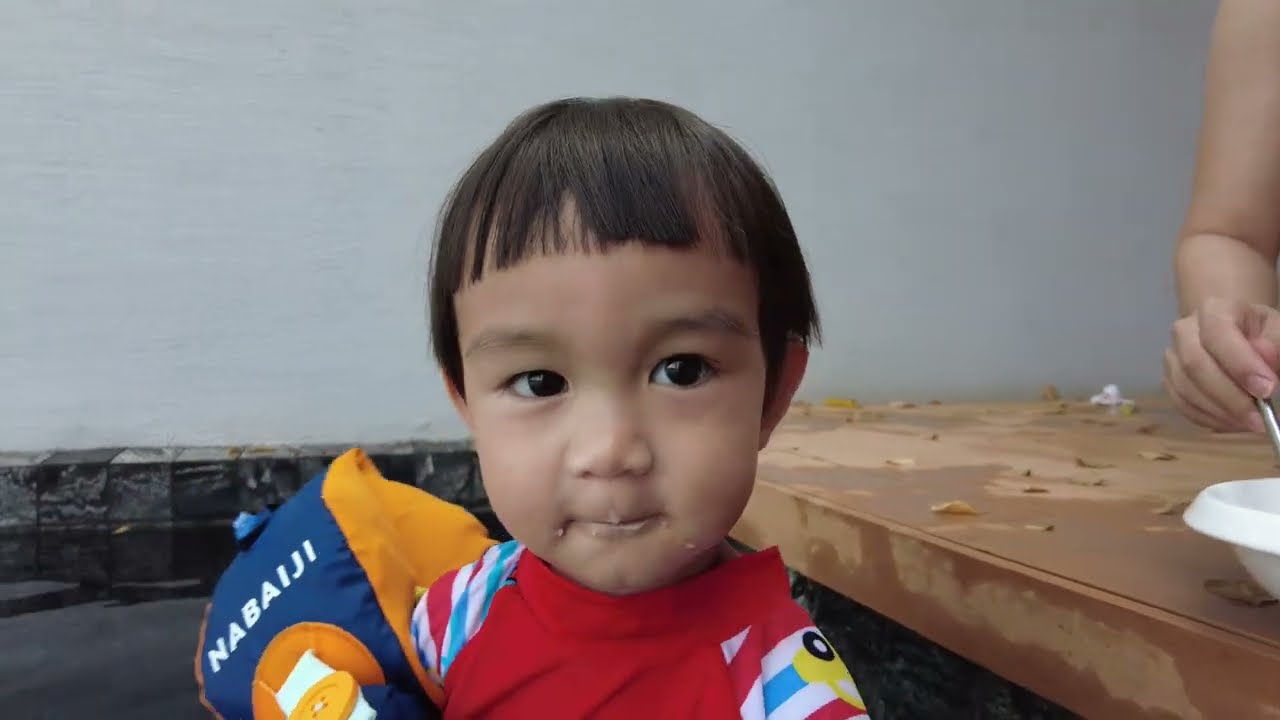This color photograph captures a close-up of a young boy, likely of Asian descent and around two or three years old, sitting beside a table. He has strikingly straight medium-length brown hair styled in a bowl cut with bangs, and his wide, dark brown eyes gaze directly at the camera. His mouth is closed, showing a hint of a smile, with traces of white cream or milk around his lips, suggesting he has just been fed. The boy is wearing a long-sleeved one-piece swimsuit in red with white and blue stripes, indicating he might be taking a break from swimming. On his right arm (the left side of the image), he sports a distinctive floatation device with navy blue in the middle and orange on the sides, labeled "NABAIJI." A woman's arm is partially visible, holding a spoon and dipping it into a white bowl on a wooden table, indicating she might be feeding him. The background shows a white wall adorned with black and gray square stones, reinforcing the outdoor, poolside setting.